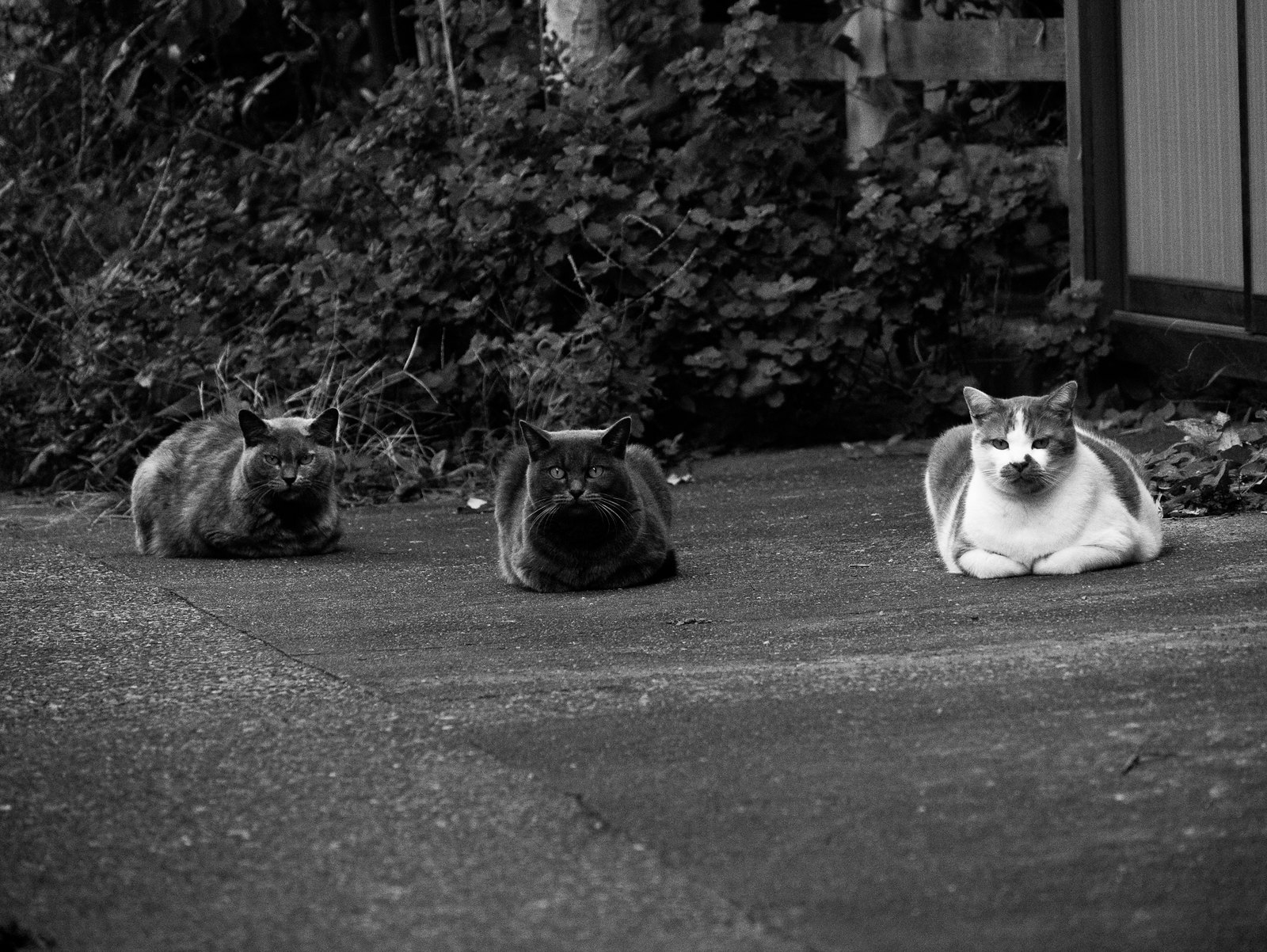This black and white photograph captures a serene moment of three cats sitting side by side, aligned horizontally in the center of the image. The scene is set on a concrete platform in what appears to be a driveway or walkway in front of a house, hinting at a residential setting. Each cat is in a loaf position with their legs tucked underneath them, and they are spaced evenly with about a foot between each other.

The cat on the left is stout, with a solid medium-gray color. It’s lying down facing roughly the 5 o'clock position, yet its eyes meet the camera, observing with a calm demeanor. The middle cat, positioned centrally from left to right, is a slightly larger black cat, frontally aligned towards 6 o'clock, also gazing directly into the lens. The rightmost cat stands out with a patterned coat of gray and white – its chest and front paws are white while its sides and face have gray markings. This cat blends the sharp contrast of its white patches with the subtler grays, adding depth to the monochrome image.

Behind the trio, there is a lush backdrop of bushy trees and shrubs, along with a wooden fence that frames the upper section of the photograph. To the right, peripheral details reveal a sliding glass door or perhaps a patio area – possibly the entrance to the home where these cats reside or are visited by their caretaker. The texture of the ground resembles tar pavement, adding to the suburban ambiance of the scene. All three cats display typical feline indifference, embodying a tranquil and aloof presence as they fix their gaze upon the photographer.